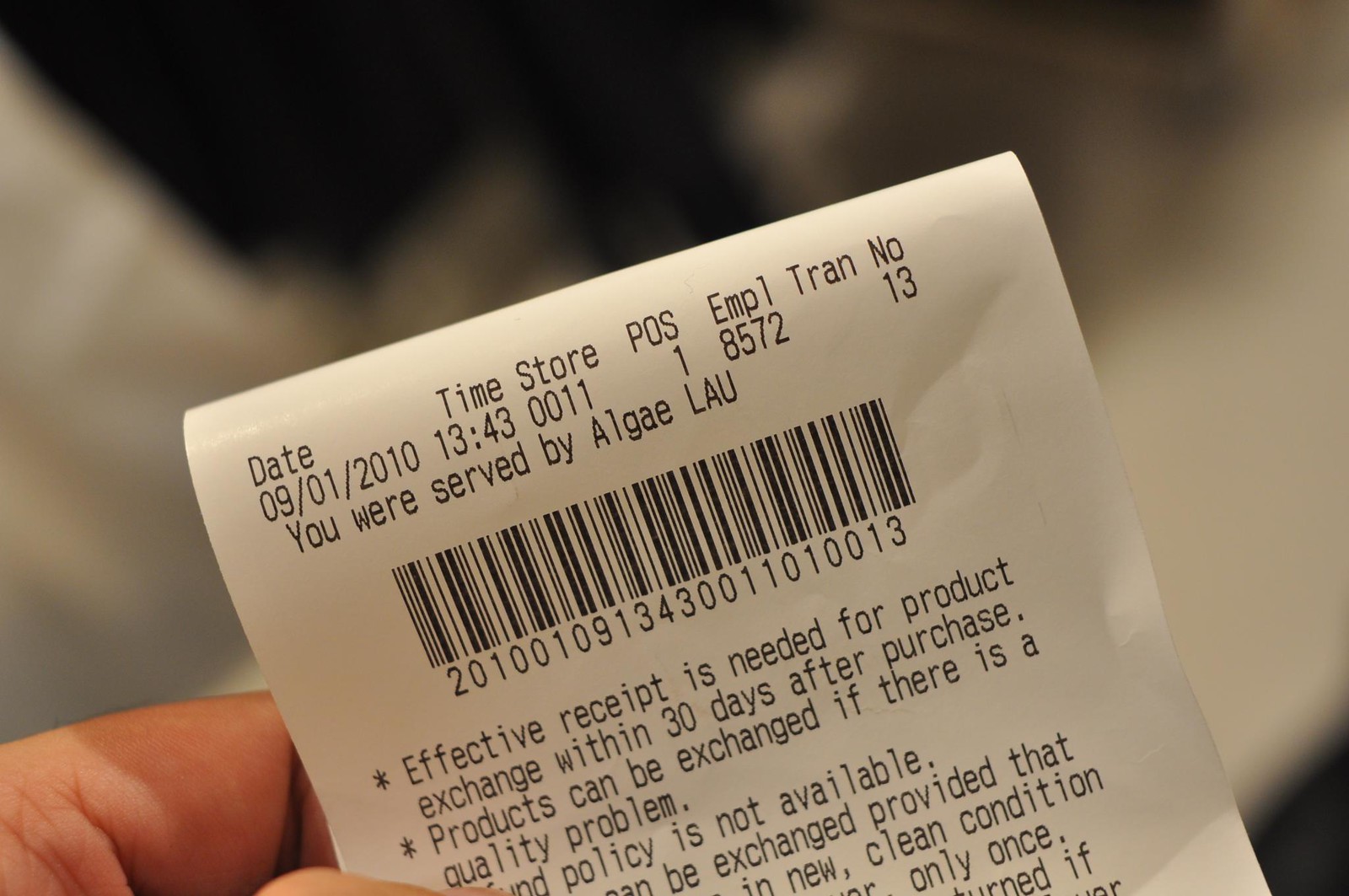In this color photograph, captured in landscape mode, a white, partially folded receipt takes center stage, tilted towards the upper left. The backdrop is blurred, highlighting the main subject. A hand, with light skin, emerges from the lower left, holding the receipt delicately between the thumb and forefinger. Key details on the receipt include the date "09-01-2010" at "13:43", store number "0011", point of sale "1", employee number "8572", and transaction number "13". Beneath these details, a long barcode is visible with corresponding numbers below. Additional text indicates store policies, though the lower portion of the receipt is cropped, obscuring some information. The receipt's top fold conceals the store's name and location, directing focus to the visible transactional details and policies printed in black ink on the white paper.